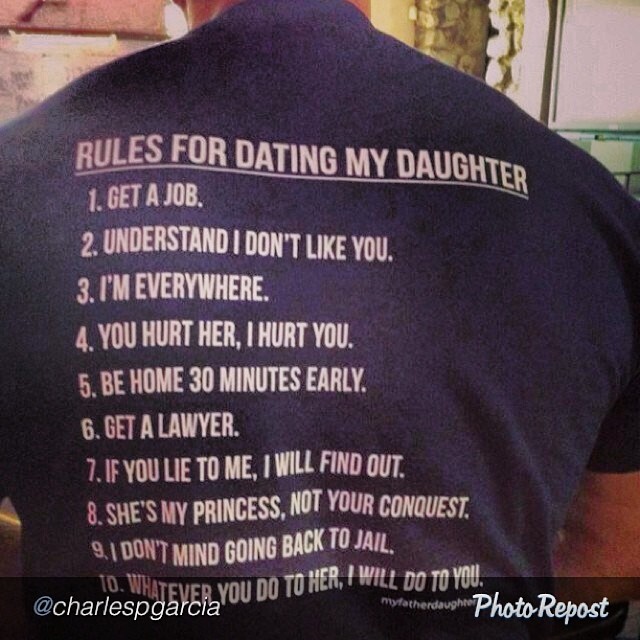This photograph captures the back of a broad-shouldered man wearing a blue, short-sleeved t-shirt adorned with white text. The shirt's text is formatted in a mix of bold and uppercase, starting with an underlined headline that reads: "Rules for Dating My Daughter." Below this headline, there is a vertical list of rules, each numbered:

1. Get a job.
2. Understand I don't like you.
3. I'm everywhere.
4. You hurt her, I hurt you.
5. Be home 30 minutes early.
6. Get a lawyer.
7. If you lie to me, I will find out.
8. She's my princess, not your conquest.
9. I don't mind going back to jail.
10. Whatever you do to her, I will do to you.

In smaller, closely spaced text, it says "Father, Daughter" at the bottom of the list. Overlaying the bottom portion of the image, there is a semi-transparent black rectangle with white text that reads "@CharlesPGarcia" on the left side and "photo repost" on the right side.